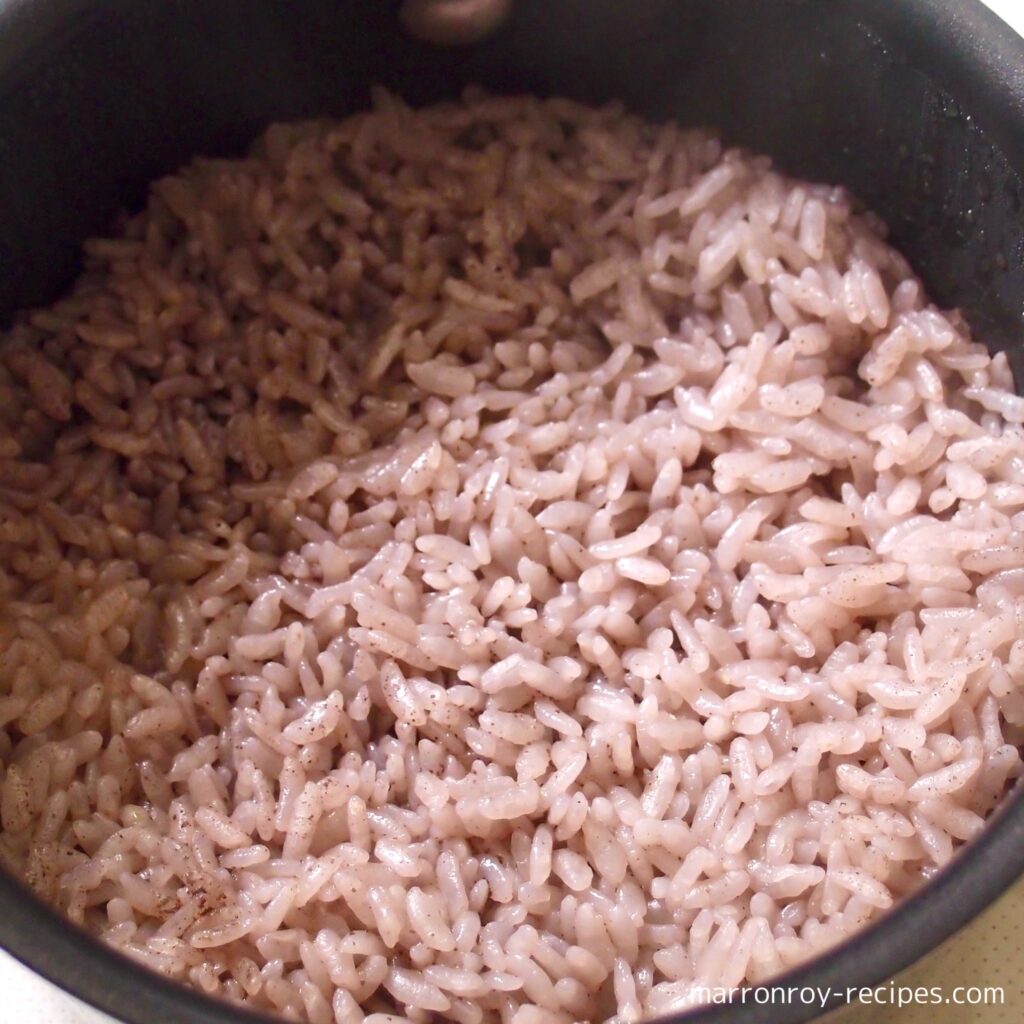This close-up image features a bowl of cooked short grain rice with a distinctive reddish-brown tint, suggesting some light seasoning distributed throughout. The dark gray bowl has a slightly moist rim, emphasizing the rice's texture. The image appears to have been taken with a filter that casts a shadow in the upper left corner, while the lower right portion is brightly lit, highlighting the rice’s wet appearance. A blurry edge of a finger is visible at the top, possibly holding the bowl. The backdrop includes a beige-patterned surface, reminiscent of a leather car seat, visible at the bottom right. A small watermark in white text reading "marenroy-recipes.com" is also situated in the lower right corner, grounding the scene in a culinary context.